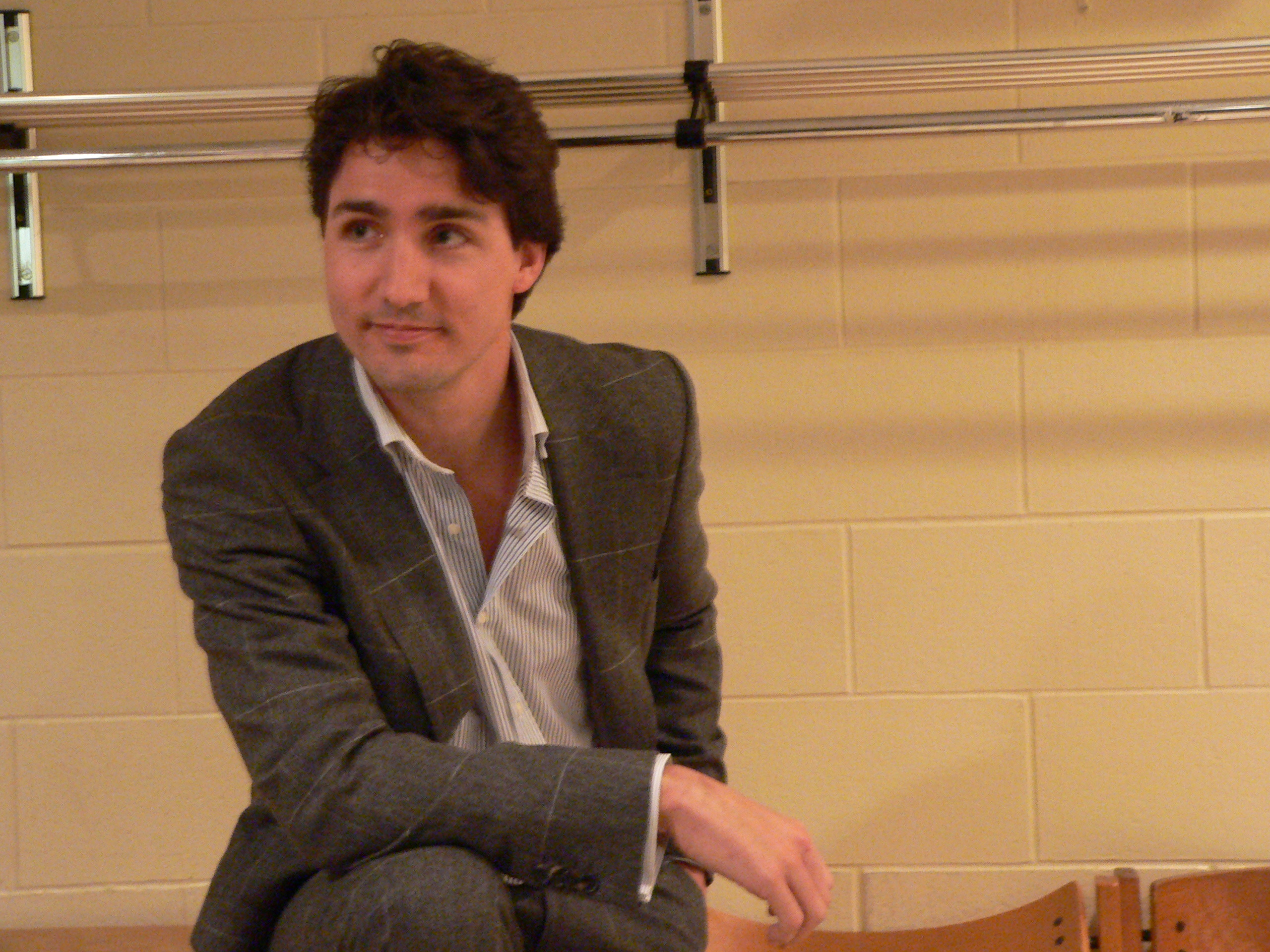The indoor photograph captures a young, Caucasian man sitting casually against a cream-colored cinderblock wall. The rectangular image, about six inches wide and four inches tall, showcases the man who has short, slightly curly brown hair and a pleasant smile. He is dressed in a medium gray, plaid dress suit adorned with horizontal light cream-colored or light gray stripes, paired with slacks. His suit jacket is open, revealing a white dress shirt decorated with thin vertical light gray or blue stripes, with its top button undone. The man’s right arm is bent at the elbow, resting on his raised knee, while his other hand is tucked into his pants pocket. In the background, extending horizontally at the top of the image, is a metal rack, possibly for luggage, attached to the cinderblock wall. To the bottom right, there is a hint of low-lying wooden chairs or a bench.